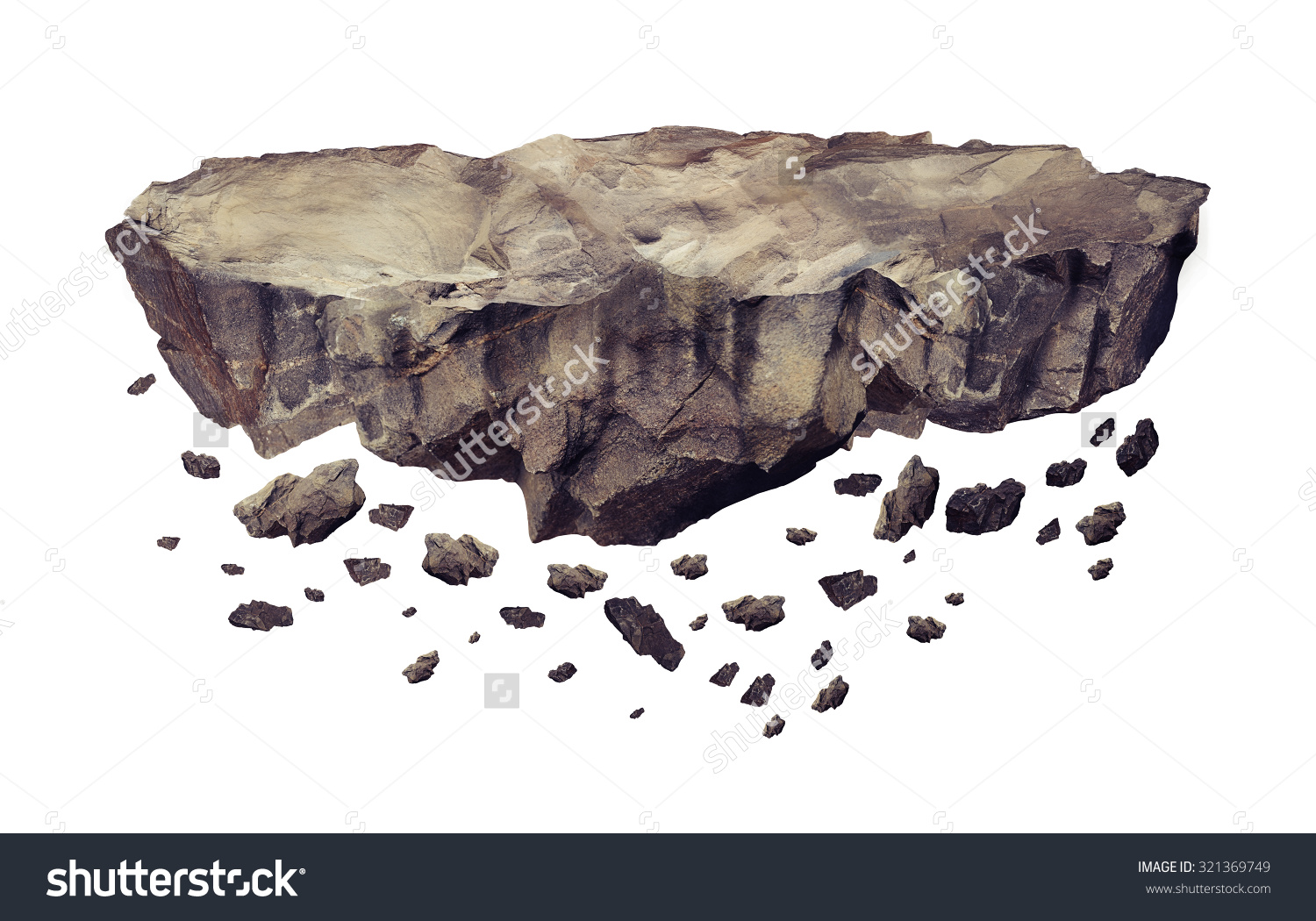The image is a detailed, watermarked stock photo from Shutterstock, featuring a realistic representation of a floating chunk of land, resembling a crumbling piece of rock or shale. The main rocky surface, rectangular in general shape, is uneven, craggy, and ridged, with jagged edges at both the top and bottom. The colors of the rock range from gray to brown and black, giving it a very earthy appearance. Beneath the large chunk are numerous smaller rocks and debris that appear to be falling off. The background of the image provides no contextual information, leaving the landmass suspended in mid-air. Watermarks consisting of "Shutterstock" in a light font are diagonally scattered across the image, with an additional light gray grid pattern watermark. At the bottom of the image, a dark horizontal band features the text "Shutterstock" on the left and "image ID 321-369-749" on the right, alongside the URL www.shutterstock.com in small white font.